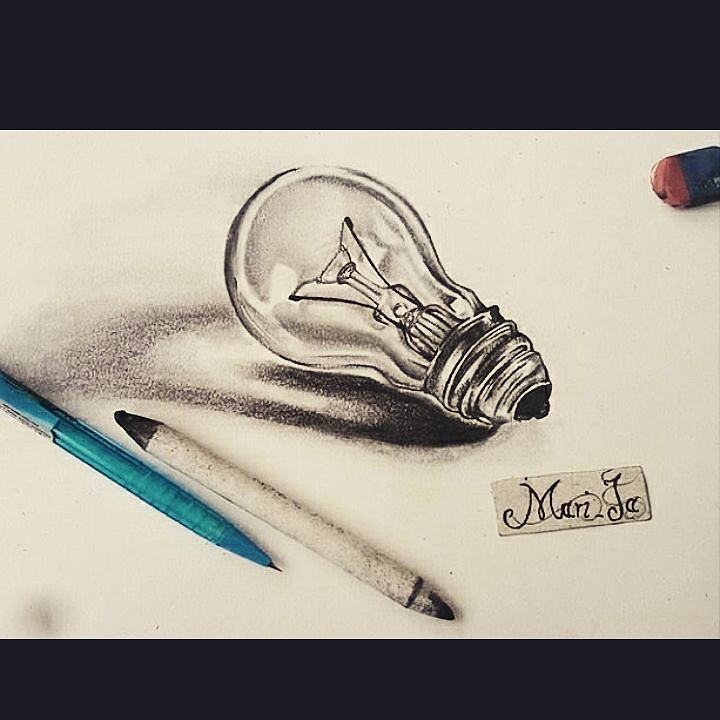The image is a rather photorealistic drawing, possibly executed in a combination of charcoal and paint. It is roughly square with thick black borders at the top and bottom, creating a pronounced framing effect. The main part of the image, set against a white backdrop, features a meticulously detailed charcoal drawing of a standard light bulb lying on its side. The threaded socket part of the bulb is positioned toward the bottom right, while the bulbous part extends to the top left. The intricately rendered filaments inside the bulb are clearly visible, showcasing expert shading techniques.

Beneath the light bulb, there is significant shadowing that extends off to the left in a curved shape, adding depth to the composition. Directly beneath and to the right of the bulb lies a two-sided charcoal drawing pencil with a white body and smudgy, used ends, also rendered in remarkable detail. Additionally, there is a blue-cased mechanical pencil towards the bottom left, its fine tip and photorealistic appearance suggesting almost palpable tactility. The tip of the mechanical pencil is cropped by the edge of the image, emphasizing a realistic depth-of-field effect.

In the upper right-hand corner of the drawing, there is a well-used artist's eraser with a dark blue wrapper and rounded, worn edges, partially veering into almost photographic realism. To the side of the light bulb is a small, darker cream rectangular piece of paper, seemingly glued onto the background. This paper bears a cursive, fancy ink signature that appears to spell "man.JA" or a similar variation, adding a personal touch to the artwork. Overall, the composition blends elements of hyper-realistic drawing with subtle, almost imperceptible photographic elements, culminating in a cohesive and richly detailed visual narrative.